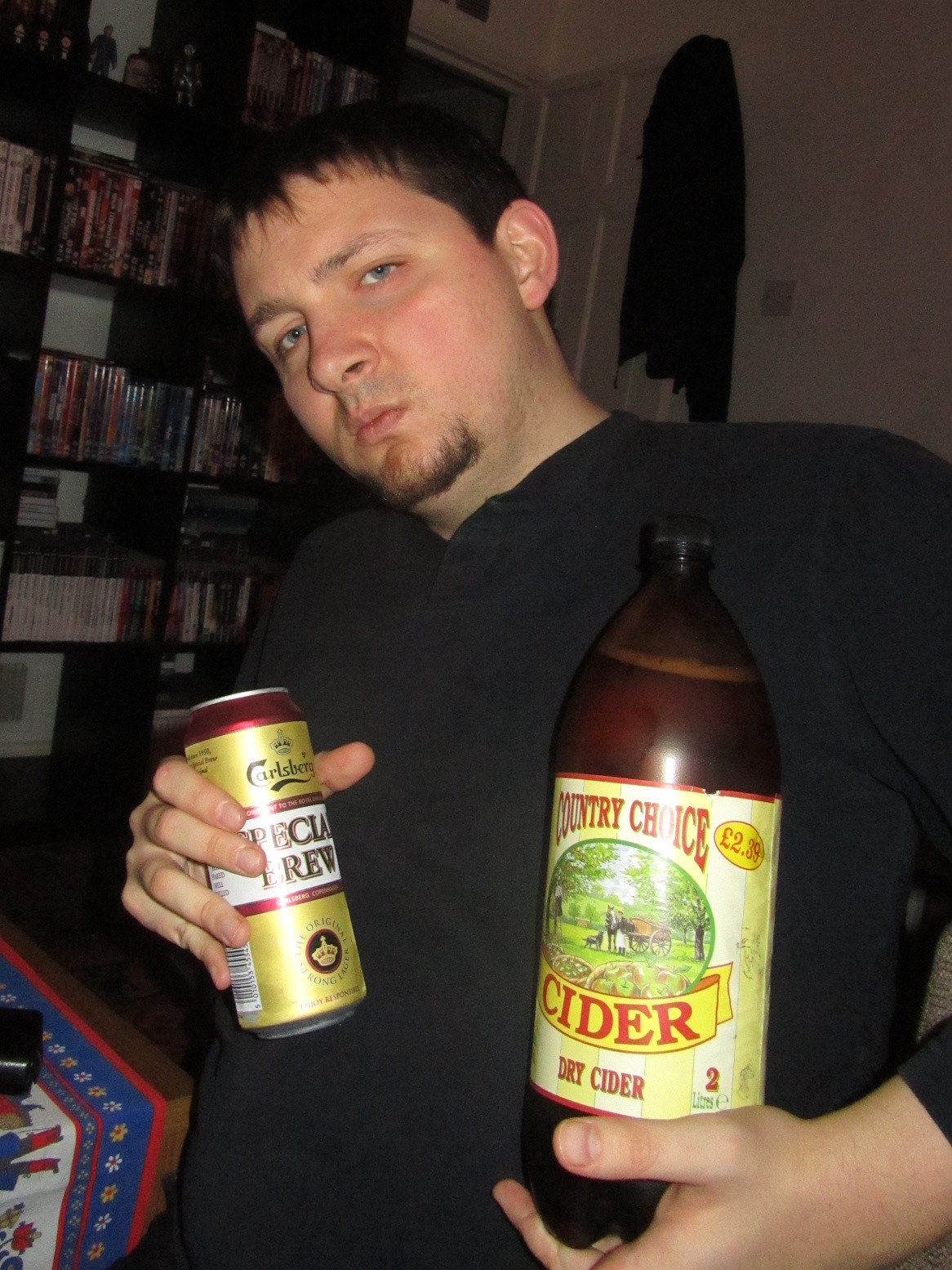The photograph captures a young man with a fair complexion and blue eyes, standing in a bedroom. He is making a serious face and has a small goatee on his chin. The man is wearing a long-sleeved black shirt. In his right hand, he holds a brown bottle with a yellow and white striped label that reads "Country Choice Cider Dry Cider," featuring a rustic image of individuals next to a wagon and wicker baskets filled with vegetables. In his left hand, he clutches a tall maroon and gold aluminum can that prominently says "Special Brew" in the middle, with additional branding details like a crown logo and the name "Carlsberg" with a wavy underline.

The room features a door that is ajar, with a dark black jacket hanging from it. To the man's left is a series of dark brown bookcases filled with various movies, books, PS3 games, and some action figures. Next to him is a light brown table that is draped with a red, white, and blue tablecloth adorned with alternating orange and white flower designs. A black object is also visible on the table. The overall setting emphasizes a cozy, lived-in atmosphere amidst a collection of personal items.